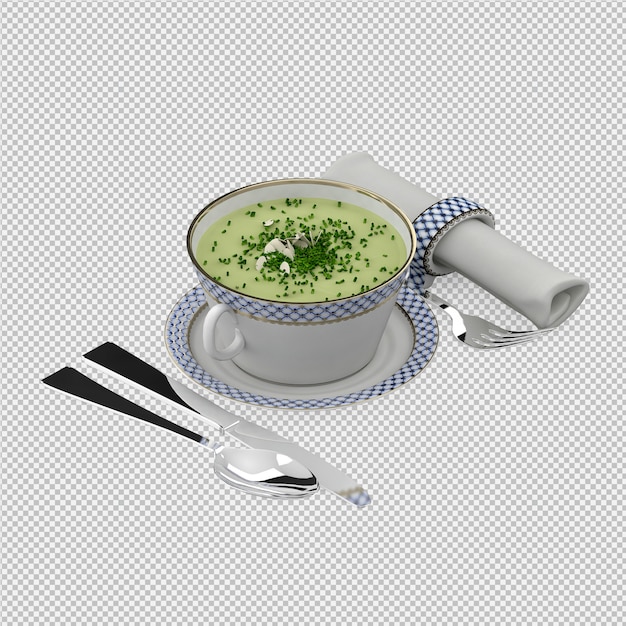This color photograph, presented in a square format, features a meticulously arranged place setting centered around a white ceramic teacup. The teacup, adorned with a blue and white diamond pattern band and a gold-lined rim, contains a creamy yellow liquid sprinkled with green specks, possibly chives or parsley, suggesting it might be a soup, though it could also be interpreted as a drink. The cup rests on a matching saucer, which sits at the center of the composition. Complementing this setup is a silver spoon and knife positioned to the left of the saucer, and a silver fork to the right. Additionally, a white cloth napkin, rolled up and secured with a blue and white patterned napkin ring, lies neatly to the right of the cup. The image has a transparent background indicated by a gray and white checkerboard pattern, highlighting the careful arrangement of the objects in a style of photographic representational realism.